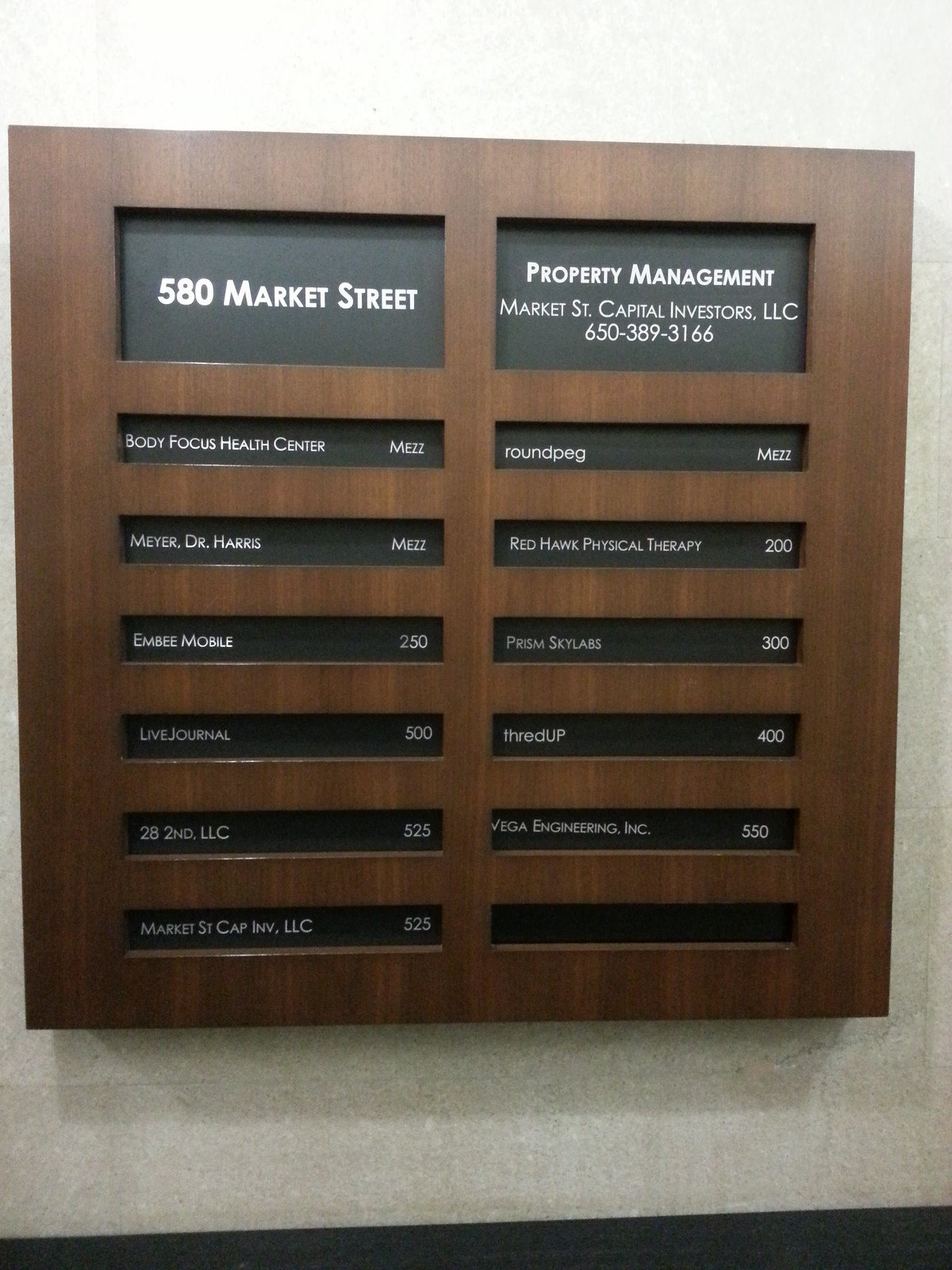The image displays an address directory board located in the lobby of a professional office building. The directory is set against a white wall and features a wooden structure with black inserts. At the top left, the board prominently displays "580 Market Street" in white letters. Adjacent to this, on the right, is "Property Management, Market Street, Capital Investors, LLC," followed by the contact phone number "650-389-3166."

Beneath this header, the board lists the tenants of the building. The left side of the board includes six entries: Body Focus Health Center - Mez, Meijer - Mez, Dr. Harris - Mez, MB Mobile - 250, Live Journal - 500, and an unspecified sixth tenant. The right side features five entries: 28 Second, LLC - 525, Market Street Cap Investment, LLC - 525, Round Peg - Mez, Red Hawk Physical Therapy - 200, and Prism Skylabs - 300. Additional tenants mentioned include ThredUp - 400 and Vega Engineering Inc. - 550, though their placement on the sides may not be explicitly stated.

This detailed directory board provides a comprehensive guide to the various businesses and their associated office locations within 580 Market Street.